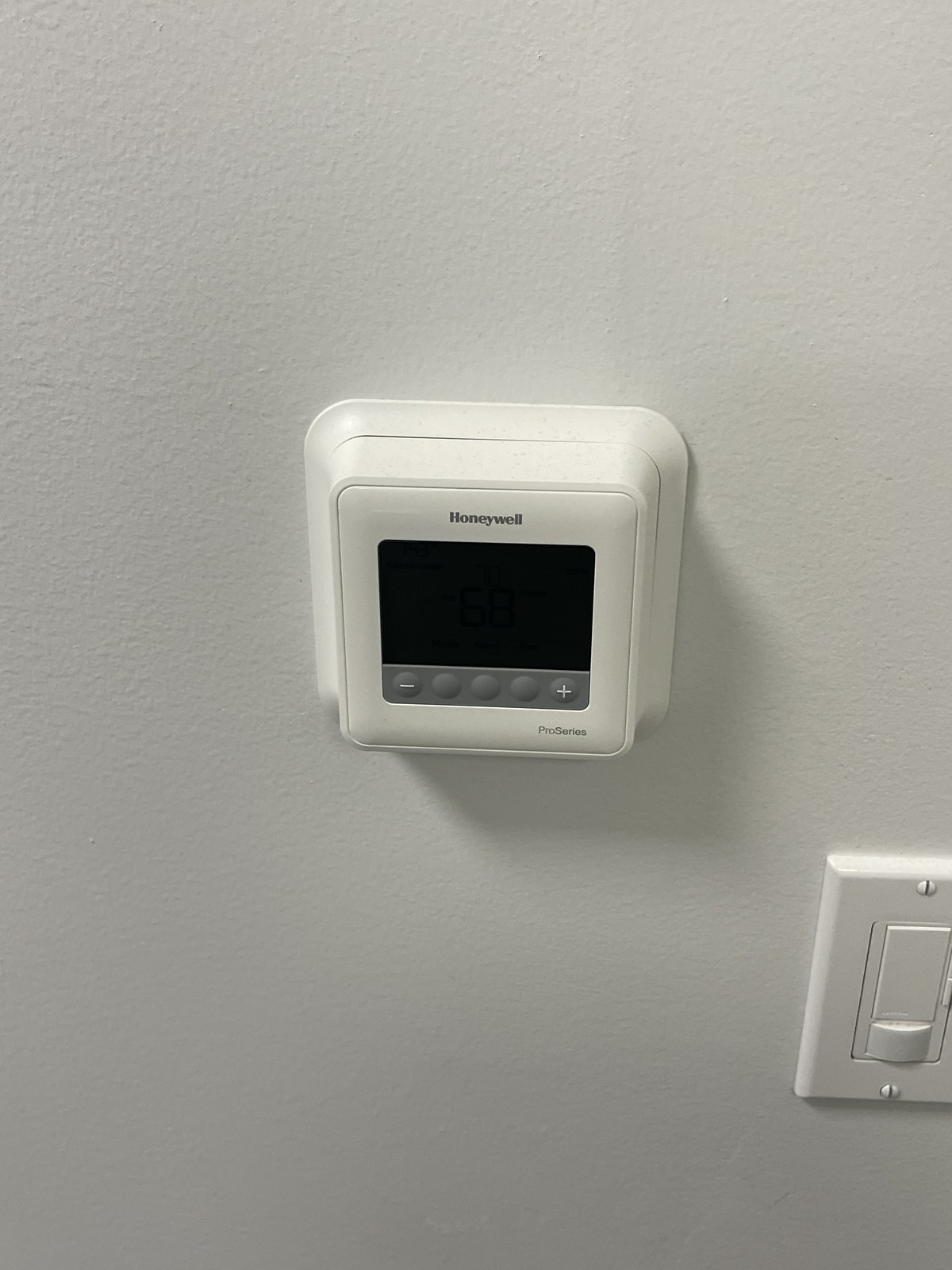This image showcases a Honeywell thermostat mounted on a white wall, possibly in a home or office setting. The thermostat is square and features a white exterior casing. Prominently displayed on the top of the casing is the Honeywell branding. The center of the thermostat has a black LED control panel, indicating that the device is currently turned off. Below the LED screen, there is a narrow gray control panel with five buttons arranged horizontally. The buttons on the far left and far right display minus and plus symbols, respectively, used to adjust the thermostat's settings. In the lower right corner of the thermostat, the model designation "Pro Series" is printed.

Additionally, mounted slightly below and to the right of the thermostat is a white push-button light switch. This switch deviates from the traditional toggle switch design, featuring a single large square push-button in its center for operation.